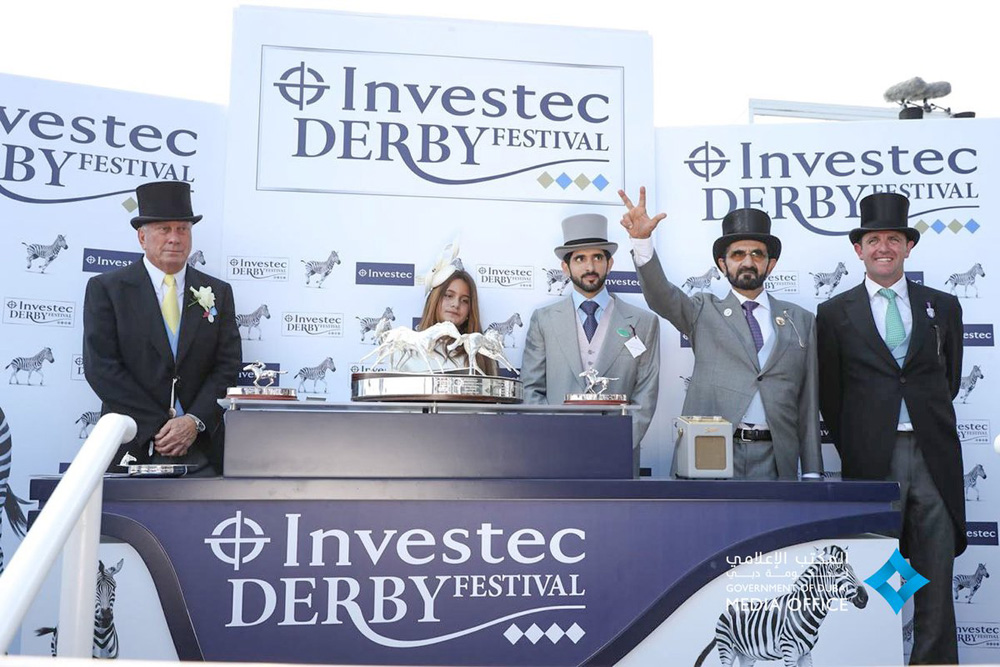This photograph captures a scene from the Investec Derby Festival. In the center, a group of five individuals stands on a stage behind a large table adorned with several shiny, silver trophies, which depict horses and riders. Four men, all dressed in suits and ties, sport top hats. The two men on the ends are in dark suits, while those in the middle wear light gray suits. One of the men in gray also has a gray hat. Beside them, a woman with long brown hair stands out with her elegant white hat. The backdrop is a prominent poster in dark blue text on a light blue background, displaying “Investec Derby Festival” thrice, across the left, center, and right sections. This backdrop features various images of horses and zebras, along with the Investec Derby's logo, complete with four diamonds in its bottom right corner. The scene includes a carousel design with several horses in front of the woman, adding a whimsical touch. A railing is visible to the left, hinting at an entrance onto the stage.